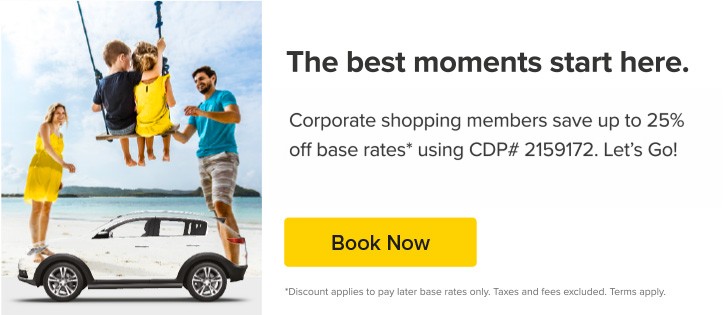This advertisement promotes a corporate shopping deal, featuring the headline, "The Best Moments Start Here" in bold text. Beneath this, smaller text highlights the offer: "Corporate shopping members save up to 25% off base rates using CDP #2159172." A prominent yellow "Book Now" button is included for immediate action. 

At the bottom of the ad, there is a disclaimer stating, "Discount applies to pay later base rates only. Taxes and fees excluded. Terms apply."

The left side of the ad features an unusual collage of images: a beach scene with a family, where the parents appear unusually tall and the kids are on swings, though the swing attachments are cut off. Below this, there is a small, semi-transparent image of a car, adding to the peculiar arrangement of visual elements.